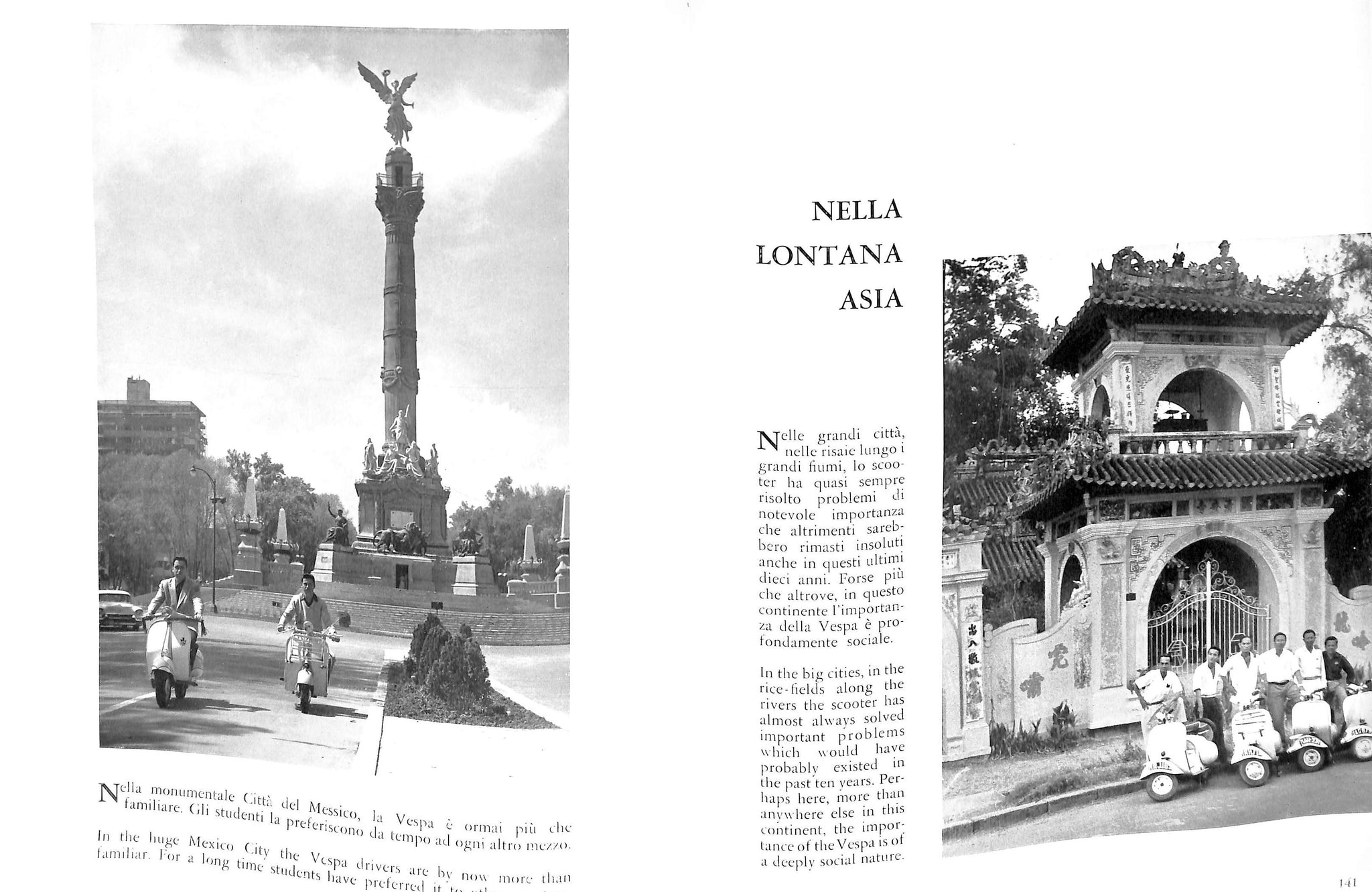An open, vintage Spanish magazine, likely about India, showcases two black-and-white photographs highlighting the importance of scooters in different cultures. The left page, labeled 140, features a bustling scene in what appears to be a major Indian city, possibly Delhi, with a large statue and people riding Vespas in front of it. The right page, numbered 141, depicts a small yet elaborately crafted temple, again with scooter riders in front. Accompanying the visuals is an article providing an English translation below; it discusses the social significance of Vespa scooters, referencing their popularity and utility in Mexico City and rural areas over the past decade. The magazine emphasizes how scooters have become essential for students and residents, solving critical transportation issues in both urban and agricultural settings.